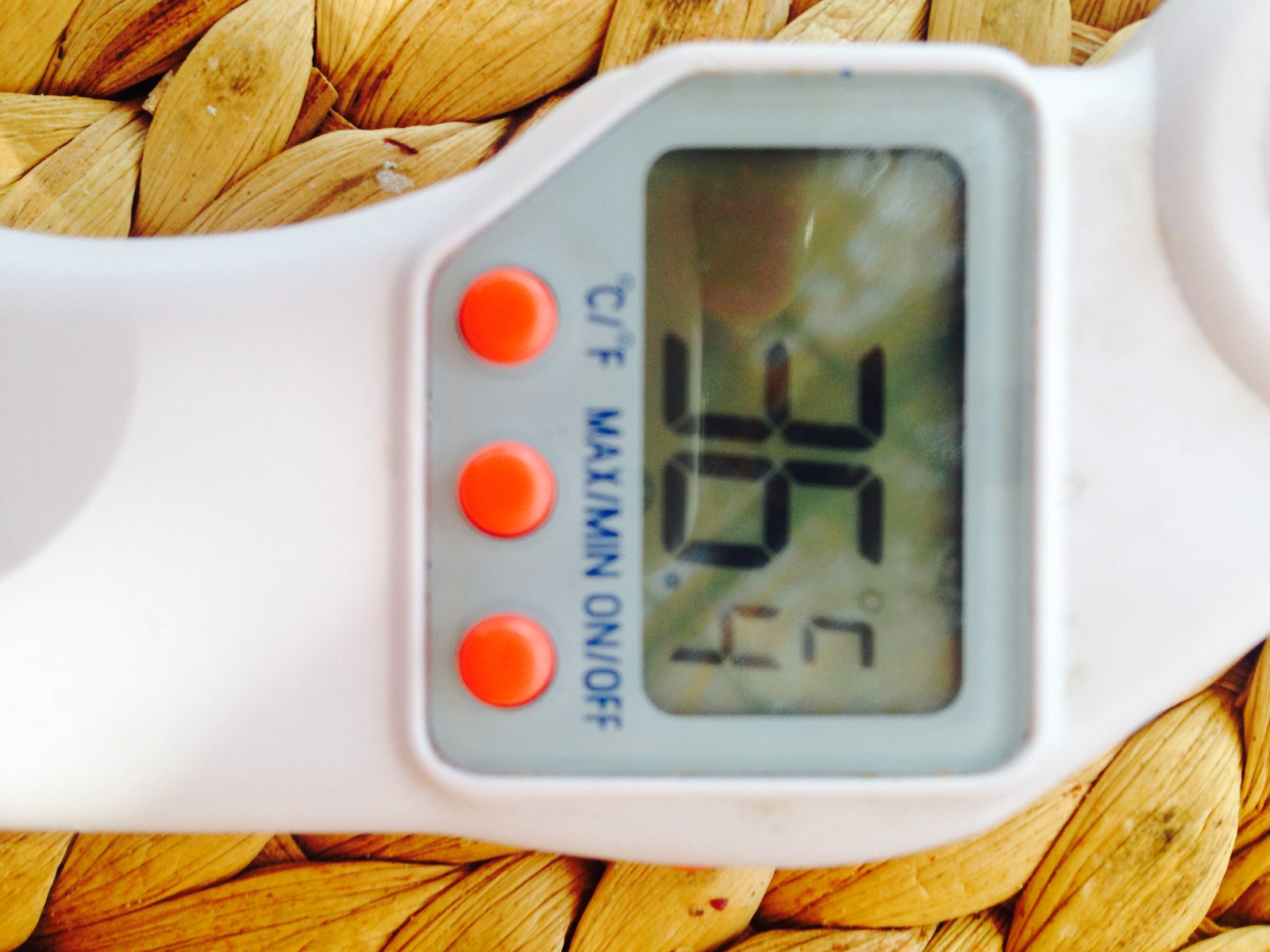A close-up image showcases a white digital thermometer prominently displaying a temperature of 36.4°C. The thermometer, which features three buttons labeled "C/F," "Max/Min," and "On/Off," appears bright and clean, though slight dirt marks are visible along the edges of its screen. Reflecting on the screen is a faint image of a finger, likely belonging to the person holding the device. In the background, a wicker basket, marred with small spots and flecks of paint, underscores the scene with its worn texture. The setting is characterized by bright, sunny conditions, suggesting the presence of numerous windows and ample natural light in the room.